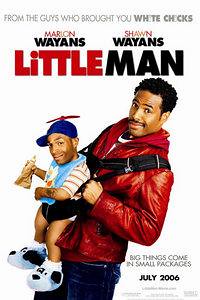The image is an advertisement for the 2006 film "Little Man," featuring actors Marlon Wayans and Shawn Wayans. The poster showcases a black actor clad in a reddish leather jacket and black jeans, leaning backward with a cheesy smile directed at the camera. He carries another black actor depicted as a child, complete with puffy dog slippers, a striped shirt, a bib, and a cap with a propeller on top. This smaller figure is secured in a baby carrier worn over the larger man's chest. The tagline "Big things come in small packages" is prominently displayed, alongside the text, "From the guys who brought you White Chicks." The film title "Little Man" and the release date "July 2006" are also clearly visible. The background of the poster is white, emphasizing the comedic visuals and playful expressions of the characters.